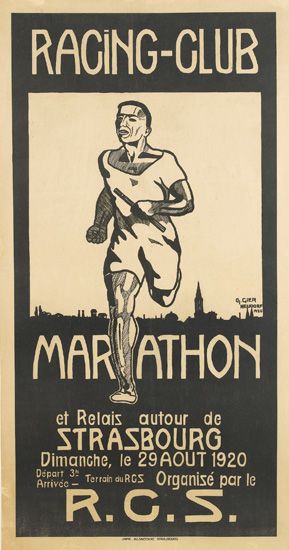This image is a vintage poster advertising the Racing Club Marathon, dating back to August 29, 1920. The poster features an old-fashioned, cream-colored background with black ink. At the very top, bold text reads "Racing-Club Marathon." Below this heading is an illustration of a man running towards the viewer, holding what appears to be a baton, symbolizing a relay race. The runner wears a white short-sleeved top and shorts, his muscular legs prominently depicted. In the background, a city skyline can be discerned, likely representing Strasbourg, France. Additional text, mostly in French, reads “Et relis a tour de Strasbourg. Die Mananche le 29 AOUT 1920,” indicating the date and location. At the bottom of the poster, there's further text that appears to be race details: "Depart: 3 Arrival: blank. Terrain du RGS Organise Parlay R.C.S." The lower part of the poster is framed in black, with white letters on the black background, and large "R.C.S." initials at the very bottom. The overall composition has a nostalgic, early 20th-century charm.